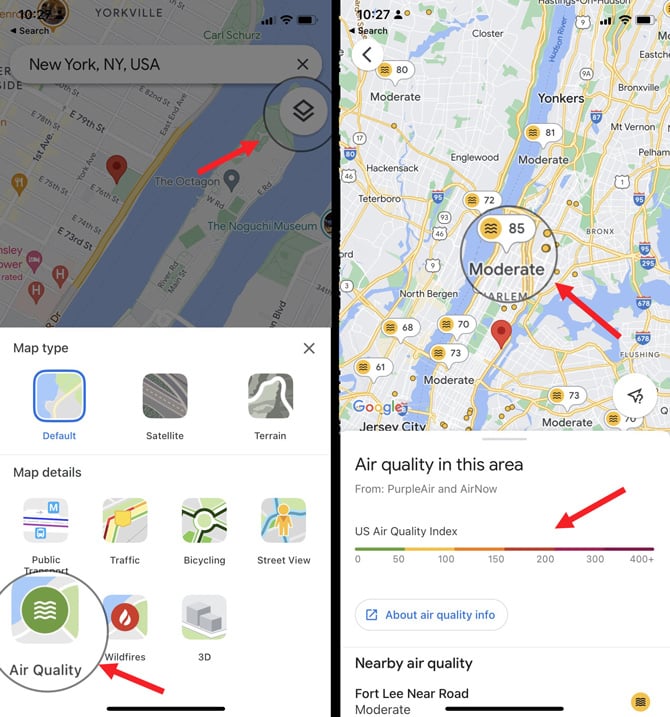On the left-hand side, the slightly gray and not very bright screenshot shows a map of New York, New York. Prominently displayed is the "Noguchi Museum" alongside blue areas representing water bodies. Yellow lines indicate slow traffic along the roads, particularly on East 73rd Street which intersects with East 74th and East 75th Streets. Below the map, there are three boxed options for map types: "default," "satellite," and "terrain," along with map details options, one of which has "air quality" circled.

Adjacent to this, another map on the right captures a central area labeled "moderate." A bubble on this map displays the number "85," suggesting this might represent an air quality index or similar metric.